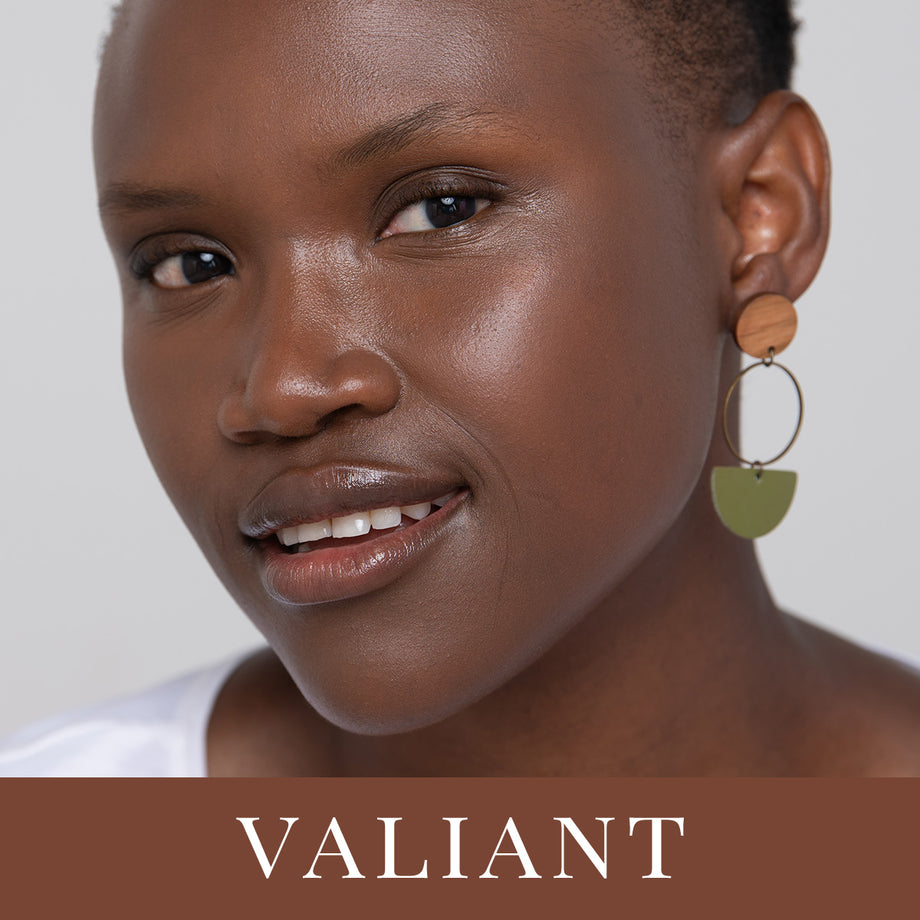The advertisement for the company Valiant features a striking image of a beautiful African-American woman with smooth, milk chocolate-colored skin, possibly in her late 20s. Her close-cropped hair draws attention to her confident gaze and bright smile, highlighted by glossy lip gloss or a brownish lipstick that complements her complexion. The woman appears in a white, round-necked shirt made of thin material, exposing her shoulders and the elegant curve of her neck.

Her face is oriented towards the left while her eyes face forward, creating a dynamic and engaging expression. She wears a bold, dangly earring in her right ear, showcasing an elaborate design: it starts with a wooden circle at the lobe, followed by a metal hollow circle, and ends with a greenish half-circle pendant. This intricate jewelry may suggest that Valiant is potentially a jewelry brand.

The background of the image is a soft light blue, adding to the serene and sophisticated ambiance of the advertisement. At the bottom, a brown banner spans the width of the photo, featuring the brand name "Valiant" in white uppercase Times New Roman font, reinforcing the professional and polished presentation of the brand and its products. This ad elegantly merges fashion and beauty, presenting the woman as a confident model perhaps symbolizing the essence of Valiant through her poised and knowing expression.